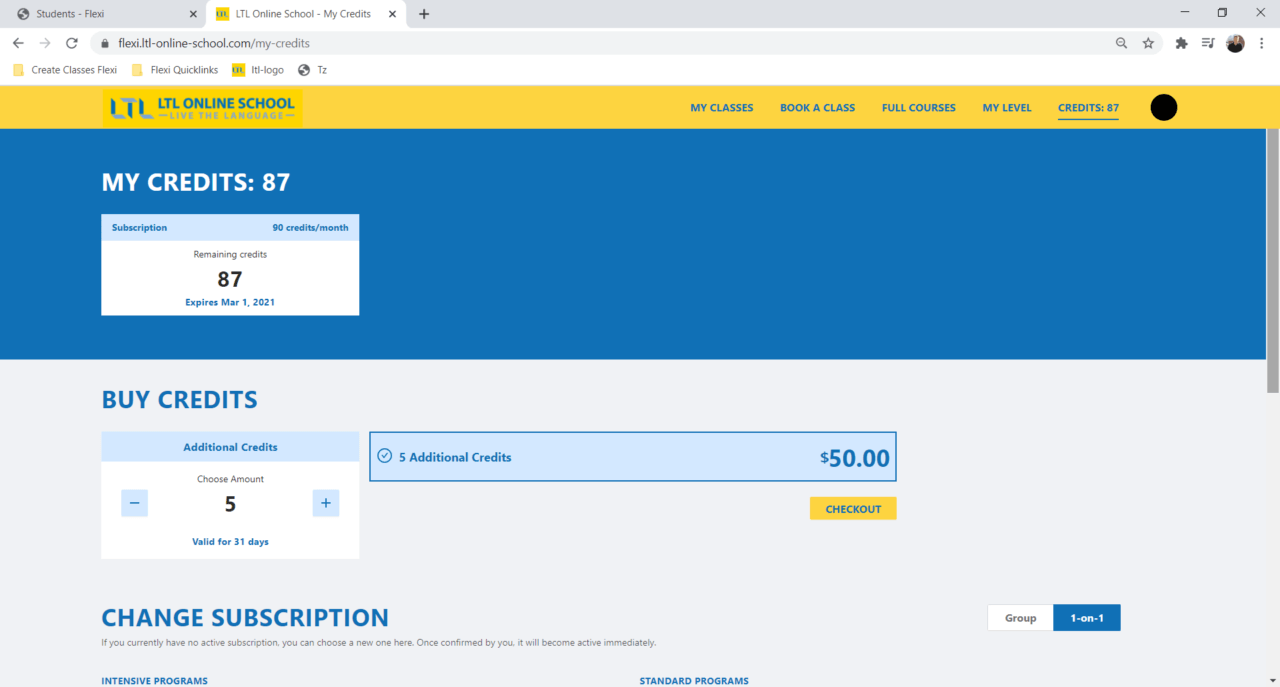The screenshot features a web browser, likely Google Chrome, open to the "ltl-onlineschool" website, a language learning platform called "Live The Language." The operating system is not visible. The user has two tabs open: one labeled "students-flexi" and the currently selected tab, titled "ltl-onlineschool-mycredits," with the URL flexi.ltl-onlineschool.com/mycredits.

At the top, the browser displays several bookmarks: "Create Classes Flexi," "Flexi Quick Links," "ITL-logo," and "TZ." 

The website’s navigation features a yellow bar with blue text. Options on this bar include "My Classes," "Book a Class," "Full Courses," "My Level," and "Credits: 87," alongside what appears to be an avatar icon.

Dominating the page is a large blue rectangle displaying "My Credits: 87." Below this are details about the user’s subscription: "90 credits a month, remaining credits 87, expires March 1st, 2021." Further down, there are options to buy additional credits, where the user can select the amount using plus or minus buttons. Five additional credits cost $50 and are valid for 31 days. There is a yellow rectangle with blue text for checkout.

Options to "Change Subscription" are provided with instructions: "If you currently have no active subscription, you can choose a new one here. Once confirmed by you, it will become active immediately." 

To the right, users can choose between "Group" and "One-on-One" classes, with "One-on-One" currently selected. At the bottom, the page has sections labeled "Intensive Programs" on the left and "Standard Programs" on the right. 

This detailed screenshot highlights the functionalities and subscription management options of an online language learning platform where credits function like tokens for classes.